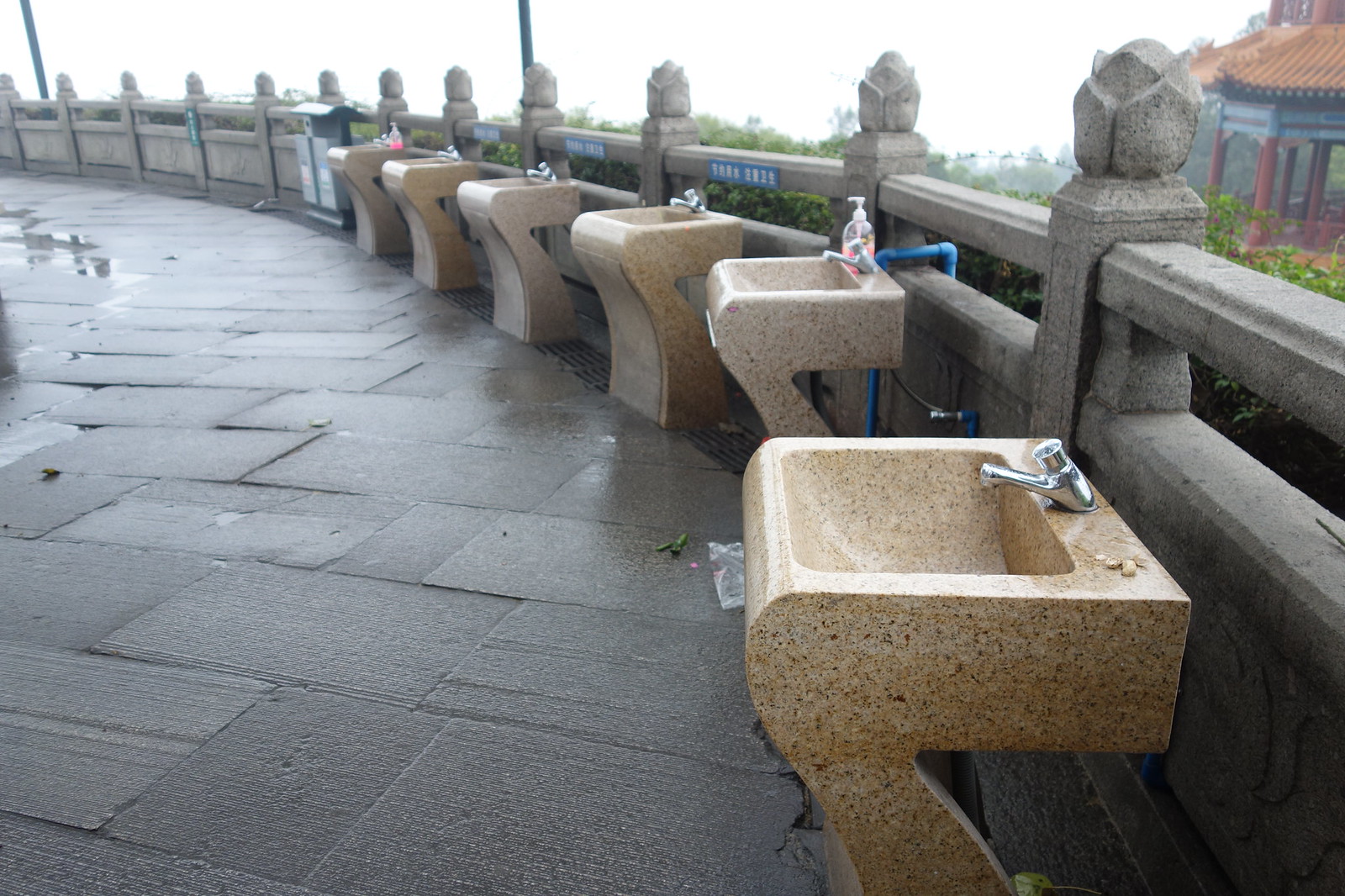In this photograph, a circular row of speckled light brown or grey granite sinks, shaped almost like backwards sevens, is arranged flush against a stone walkway. Each elegant sink is fitted with a single silver tap. The stone walkway itself is bordered by a stone railing adorned with posts featuring ornate embellishments that resemble rosebuds. Behind the railing, the tops of lush green trees are visible, suggesting the walkway is elevated. In the top right corner of the image, a partial view of a red and gold pagoda adds a touch of cultural richness, hinting that the location might be in Asia, possibly China or Japan. Blue signage is affixed to the stone railings, further indicating the walkway’s likely Asian origin. The pagoda, with its orange roof, blue painting, and reddish-brown uprights, overlooks a scene that combines functional architecture with natural beauty, creating a unique and picturesque environment.